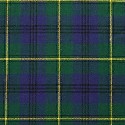The image depicts a close-up of a small piece of fabric featuring a detailed, plaid pattern. Dominated by forest green and deep cobalt blue hues, the fabric showcases a checkered design. Thin yellow lines crisscross to form a grid, creating multiple squares. Within these squares, there are vertical black pinstripes running on top of the blue backdrop. Each square also contains a purple section that contrasts with the green parts, intersected by black and yellow lines. The intricate pattern repeats throughout the fabric, potentially indicative of a Scottish kilt or similar textile. The detailed, woven texture suggests a high-quality, knitted construction.